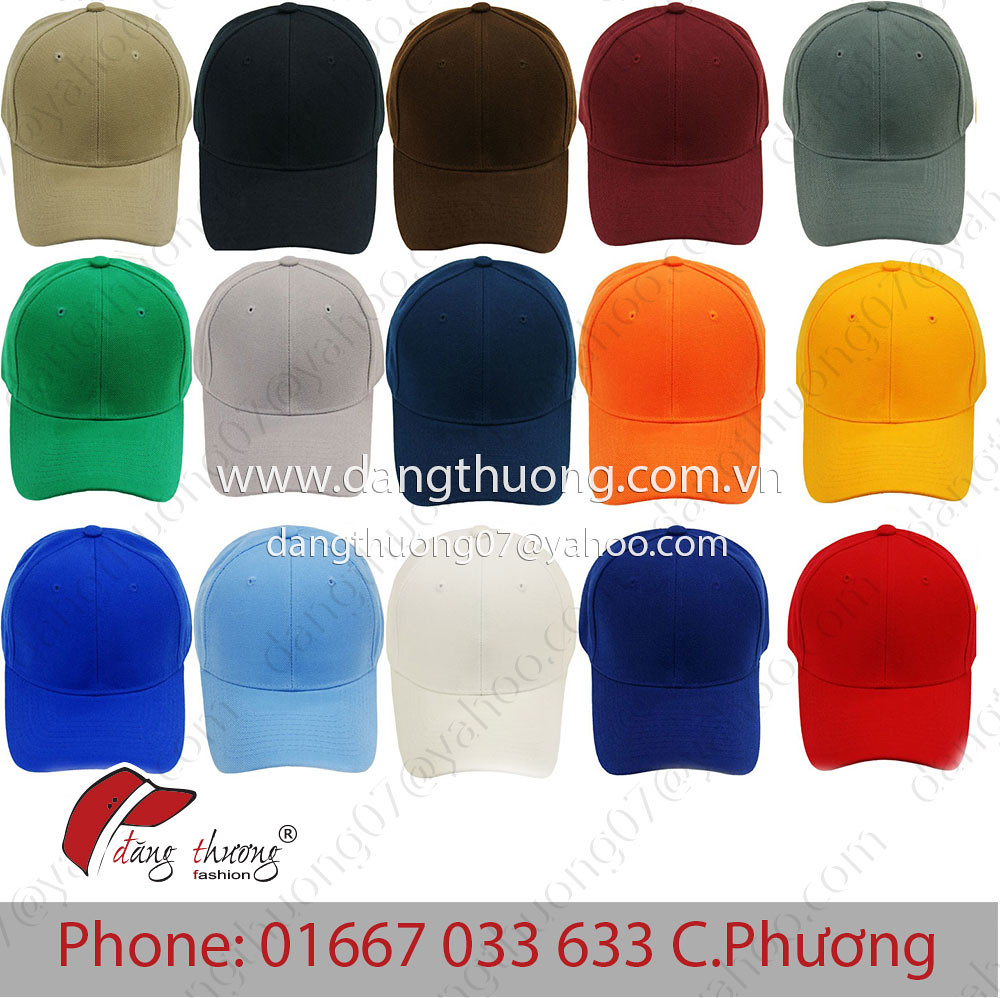This image is a detailed catalog page showcasing 15 baseball caps arranged in three rows of five, featuring a wide array of colors including beige, black, brown, maroon, turquoise, green, blue (with various shades such as electric blue, light blue, and baby blue), white, midnight blue, bright yellow, bright orange, bright red, and cream. In the center of the image, in white lettering, it prominently displays the website www.dangthong.com.vn. Below it, the email address d-a-n-g-t-h-u-o-n-g-o-7 at yahoo.com is listed, along with another mention of dangthong07.com. Multiple watermarks reading "dangthong fashion" are scattered throughout the image. The bottom-left corner features an offset ball cap image with "dangthong fashion" inscribed below it, followed by a gray box containing red numbers and lettering for the contact phone number 01667-033-633-c.phoung.